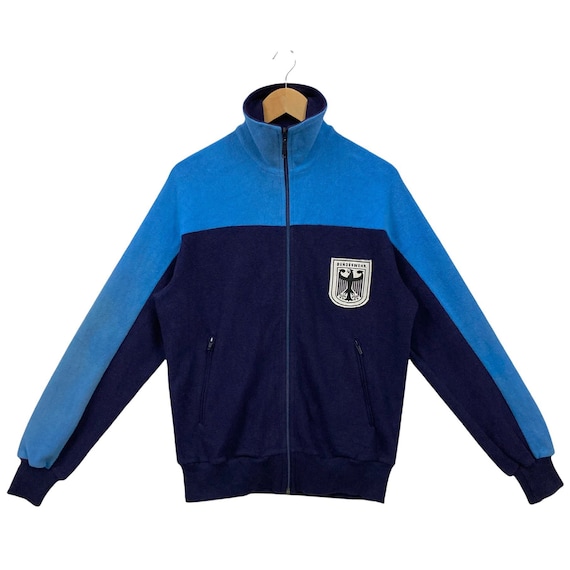In the image, there is a jacket, hanging neatly on a wooden hanger with the hook visible above the neck area. The jacket features a stylish, zippered design, fully zipped up the front. The upper portion of the jacket, extending from the chest up through the arms, is a light blue color, while the lower section and the wrist areas transition into a darker navy blue. The garment includes two front pockets, both secured with zippers. On the right breast, there's a distinctive white patch with a curved bottom edge, featuring a black symbol that resembles a bird; above this patch, there’s some unreadable text in black. The jacket appears to be appropriately sized for a teenager or a smaller adult, although it does not look to be extra large.